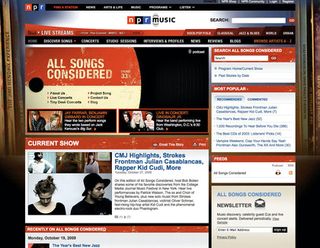A small image showcasing the NPR Music website. The image prominently features the "All Songs Considered" section, highlighting various articles and a curated list of songs. Among the articles, there is a feature on CMJ highlights, which includes notable mentions of Strokes frontman Julian Casablancas and rapper Kid Cudi, among others. Although the article's text appears too small to read clearly, there's an associated image or headline next to it. On the right sidebar, additional information and options are available, including an option to subscribe to the NPR Music newsletter.